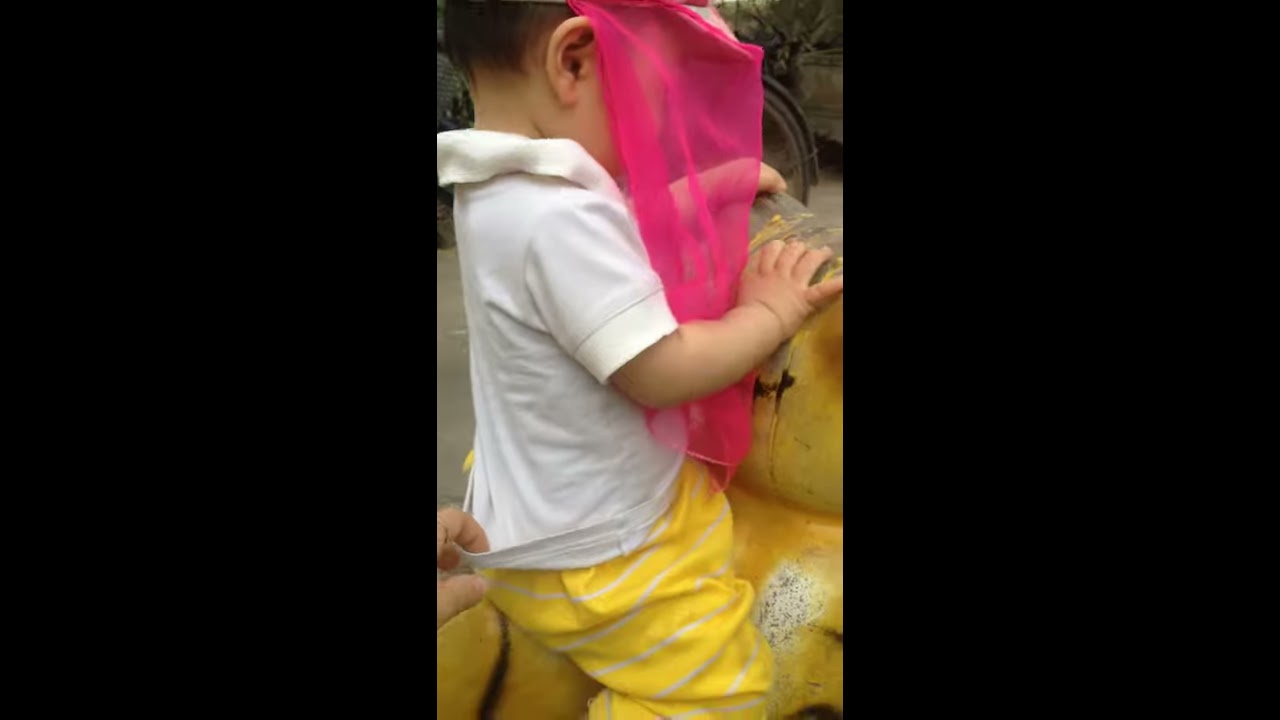Set outdoors, this detailed center panel of a triptych features a toddler, likely of Asian descent, whose face is obscured by a large pink visor or a netting hat, possibly intended for mosquito protection. The child, dressed in a short-sleeve white t-shirt and yellow pants with white stripes, sits atop what appears to be a toy or ride-on animal. An adult's hand is seen gripping the back of the child’s shirt, ensuring he remains secure on the toy. His small hands rest on the yellow figure he’s riding. In the background, there are bushes, and the black coloring of the side panels frames the scene with no accompanying text.